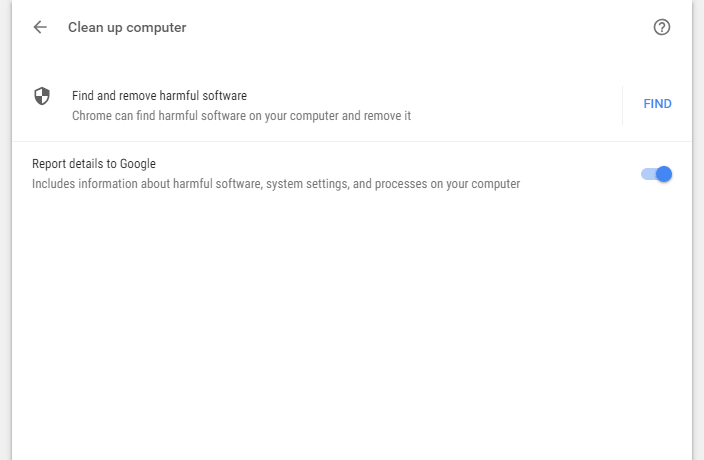The image displays a "Clean up computer" menu screen from Google Chrome. In the top-left corner, there is a back arrow icon followed by the text "Clean up computer." On the far right, there is an icon of a circle with a question mark inside it, likely indicating a help or support option. Below this, there is a shield icon, predominantly white with black sections in the bottom-left and top-right corners, symbolizing security.

Adjacent to the shield icon, the bold text "Find and remove harmful software" is highlighted. Underneath, a descriptive sentence in lighter text reads, "Chrome can find harmful software on your computer and remove it." To the right of this text, the word "FIND" is displayed in full capital letters and blue text, indicating an actionable button.

Further down, the text "Report details to Google" appears in black followed by a more detailed explanation: "Includes information about harmful software, system settings, and processes on your computer." Next to this description, there is a toggle bar with a circle on it. The bar is light blue, and the circle is a darker shade of blue, indicating that the reporting feature is currently activated.